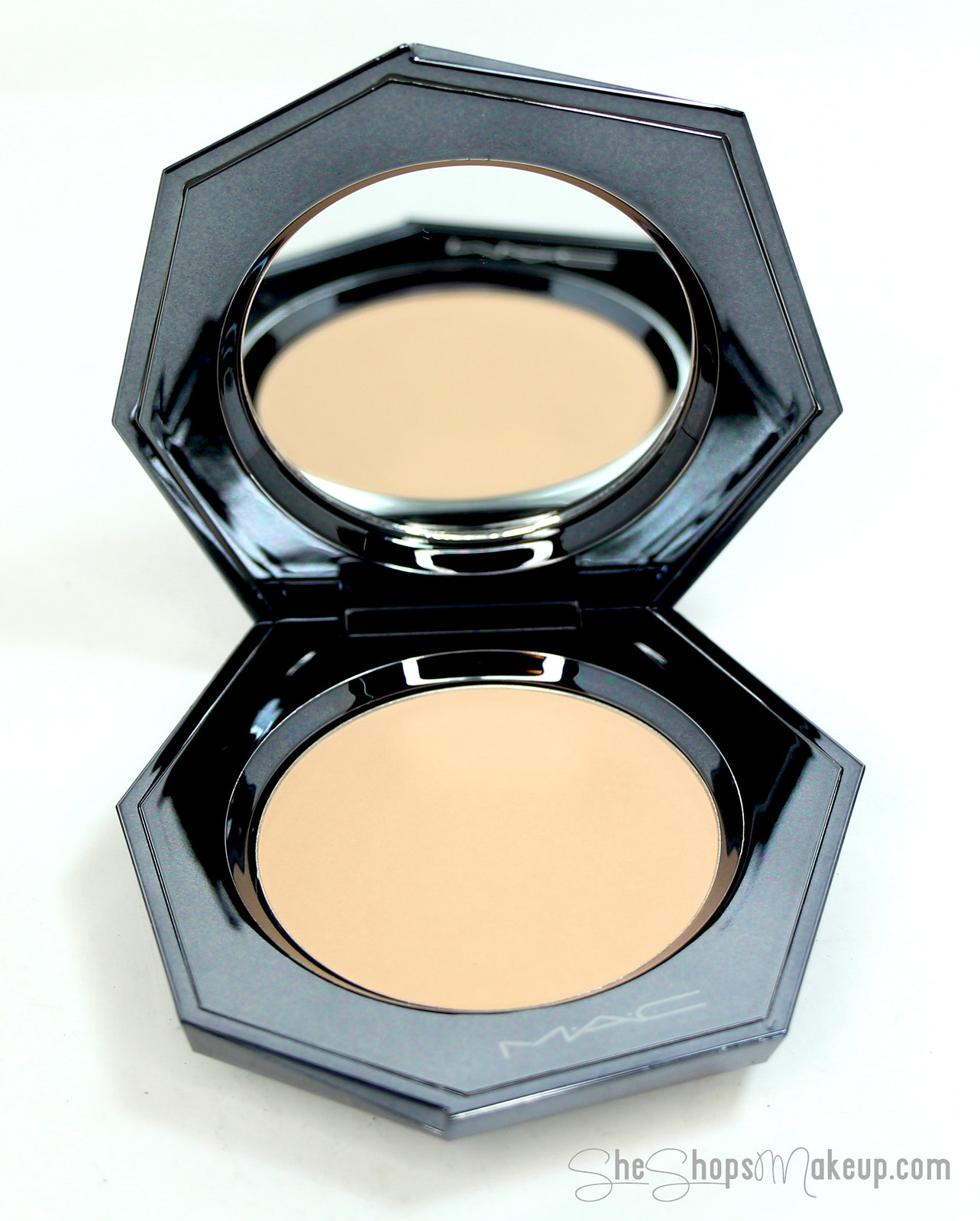The image displays an open makeup compact on a white surface, with a white background. The compact has a unique hexagonal shape and features a metallic, dark charcoal gray exterior. The interior of the compact lid houses a round mirror, which reflects the light beige, peachy-beige makeup contained in a round pan at the base. The makeup compact prominently displays a MAC logo along the bottom part. Additionally, there is a watermark in gray text, "SheShopsMakeup.com," positioned in the bottom right corner, lending an added touch of professional branding. The compact exhibits a sleek, modern design with visible drop shadows adding depth to the image.